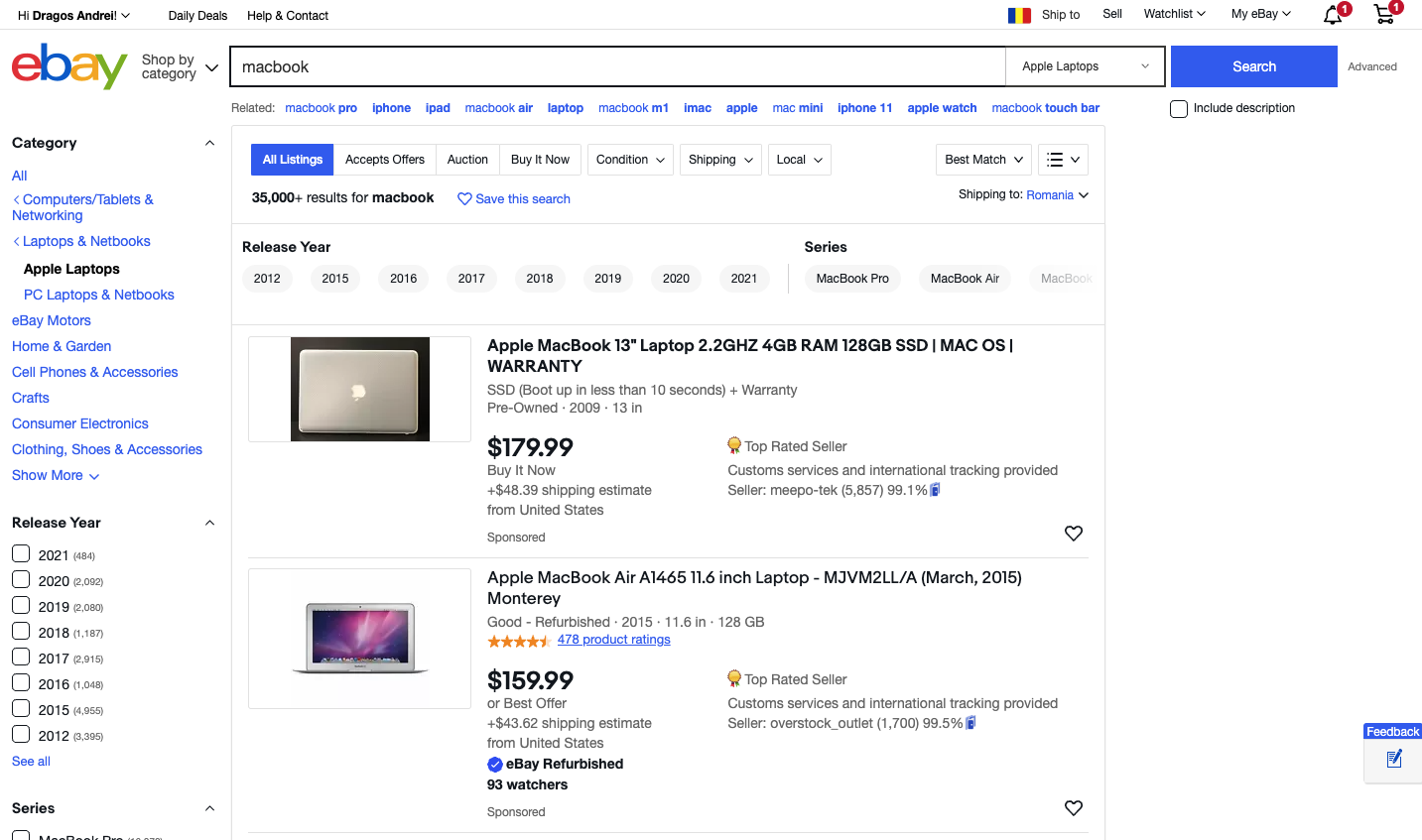Screenshot of an eBay webpage:

At the top of the screenshot is a white background with black text on the left side reading, "Hi Dragos Andreal," followed by menu options, "Daily Deals," "Help & Contact." On the right side, there's a flag with blue, yellow, red, and black colors beside menu terms, "Ship to," "Sell," "Watchlist," and "My eBay." The bell icon and shopping cart icon both have a notification badge with the number '1'.

On the left, the logo "eBay" is displayed in a mix of red, blue, yellow, green, and black. Below it, there are options for "Shop by category" and a search bar where "Macbook" is typed in. To the right of the search bar is a blue "Search" button with white text. Below this bar are trending search terms in blue text like "Macbook Pro," "iPhone," "iPad," "Macbook Air," "Laptop," "Macbook M1," "iMac," "Apple," "Mac Mini," "iPhone 11," "Apple Watch," and "Macbook Touch Bar."

Further down on the page, options to filter listings are available: "All Listings," "Accept Offers," "Auctions," "Buy It Now," "Condition," "Shipping," and "Local." On the left side, there is a blue category list titled "All Categories" with subcategories related to Mac products, including a filter for "Release Year" ranging from 2021 to 2012.

Displayed in the results is an Apple MacBook 13-inch laptop featuring a white Apple logo. The listing details include "2.3 GHz, 4 GB RAM, 128 GB SSD, macOS" priced at $179.99 with "Buy It Now" and $48.38 shipping from the United States. Another listing shows an open MacBook Air priced at $160 with $43.60 for shipping.